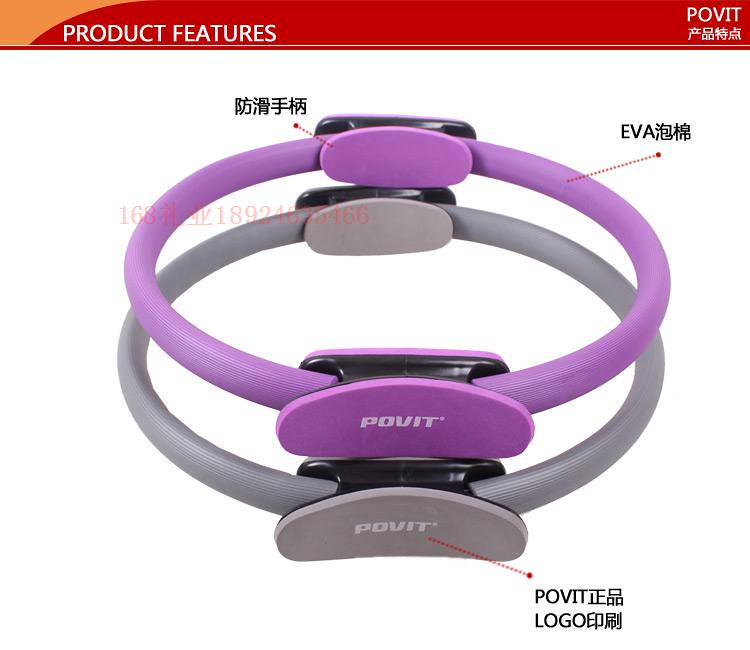The image displays a full-color photograph with a plain white background and a prominent header at the top. The header is predominantly red, with a small portion on the left transitioning into orange, finished with a thin white pinstripe at the bottom. It spans almost the entire width of the image, featuring large white, bold, capitalized letters stating "Product Features" on the left. On the right side of the header, it reads "POVIT" in white, followed by some Asian characters beneath it.

Below the header, the image showcases two circular wrist bracelets or possible fitness bands, one positioned above the other. The upper bracelet is lavender or purple and consists of two sections, each containing black clips that hold sensors. The clips bear the "POVIT" logo in white print. The lower bracelet is gray and has a similar design, also featuring black clips with the "POVIT" logo. 

Various arrows point to specific features on the bracelets. One arrow highlights the sensor on the purple band, labeled "EVA" followed by Asian writing. Another arrow from the bottom points to the "POVIT" logo, again followed by Asian characters. Additional red print on the left side of the image starts with the number "168," proceeding into Asian characters and ending with a series of digits "18924635466."

The detailed description and annotations suggest these bracelets have specialized components, likely indicating product specifications or features in the Asian text.